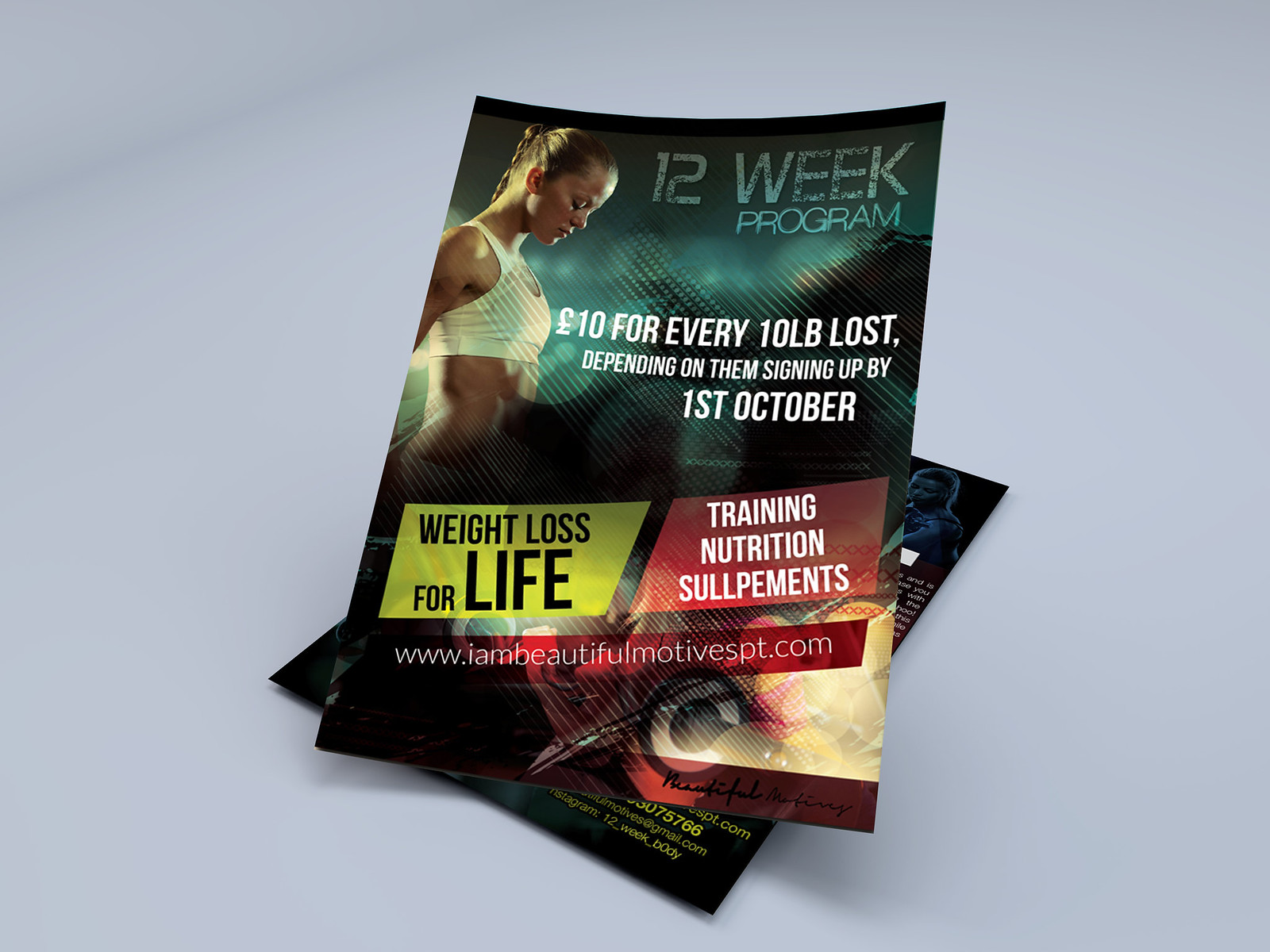The image shows two overlapping flyers set against a light blue background. The top flyer prominently features a woman in a sports bra, looking down with her hair pulled back. On the right side of her image, large text announces a "12-week program" with a special offer: "$10 for every 10 pounds lost," contingent upon signing up by October 1st. Below this, in white letters, it further details “weight loss for life” in a yellow box and “training, nutrition, supplements” in a red box. At the bottom center of the flyer, the website www.iambeautifulmotivespt.com is displayed. The second flyer is partially visible underneath, positioned at an angle, showing a person in the top right corner and some contact information in the bottom right corner.